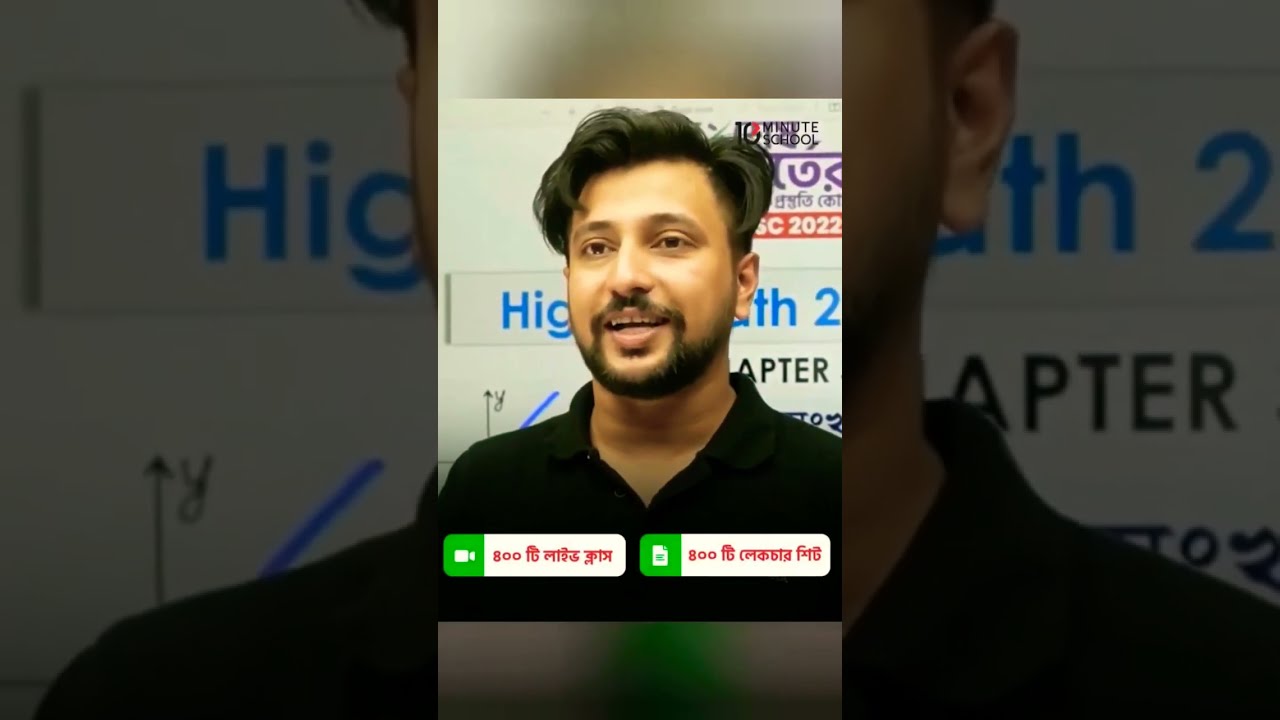In this image, there is a central vertical rectangular strip containing a photograph of a man of Indian descent with brown skin and black hair. His hair is relatively short and parted on the left, complemented by a full beard and mustache. The man is wearing a black button-down shirt without a tie. His mouth is open as if he is speaking or smiling, suggesting he is communicating something.

Behind the man, there is a poster displaying some text, one part of which includes a graph with blue elements and text that is partially obscured by his head. The text appears to be in Indian script, indicating the setting may be related to Indian culture or language. Additionally, there are horizontal green strips both above and below the central photograph, which are blurred and resemble the zoomed-in background of the same image.

At the bottom of the central image, more text can be seen, also in a foreign language, possibly Indian. It appears there are clickable icons below this text, one resembling a camera and another for a note pad, suggesting additional digital content like a PDF or video might be accessible.

The overall scene suggests that the man might be addressing an audience, possibly discussing financial matters or mathematics, given the graphical content in the background. The detailed context, including his appearance, attire, and the setting, portrays him as a speaker or lecturer, potentially a math teacher or an expert in a particular field engaging with his audience.